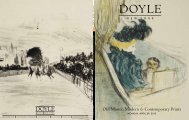The image features two small, side-by-side drawings, both notably blurred and difficult to discern. The left drawing predominantly showcases a scene that vaguely resembles three black and white horses racing, accompanied by spectators in the stands. Beside it, a green curtain is faintly visible. The right drawing, under the title "DOLE" printed in bold, capitalized letters, depicts a woman standing in front of a testimonial stand in a court setting. This woman is donned in a black furry hat and coat. Surrounding her are several indistinct animals, likely horses, with a backdrop of plants. Despite the lack of clarity, it appears that this right image may also resemble or relate to the cover of a book. The style of the drawings hints at a medium possibly involving colored pencils, characterized by muted tones and a cartoonish simplicity.